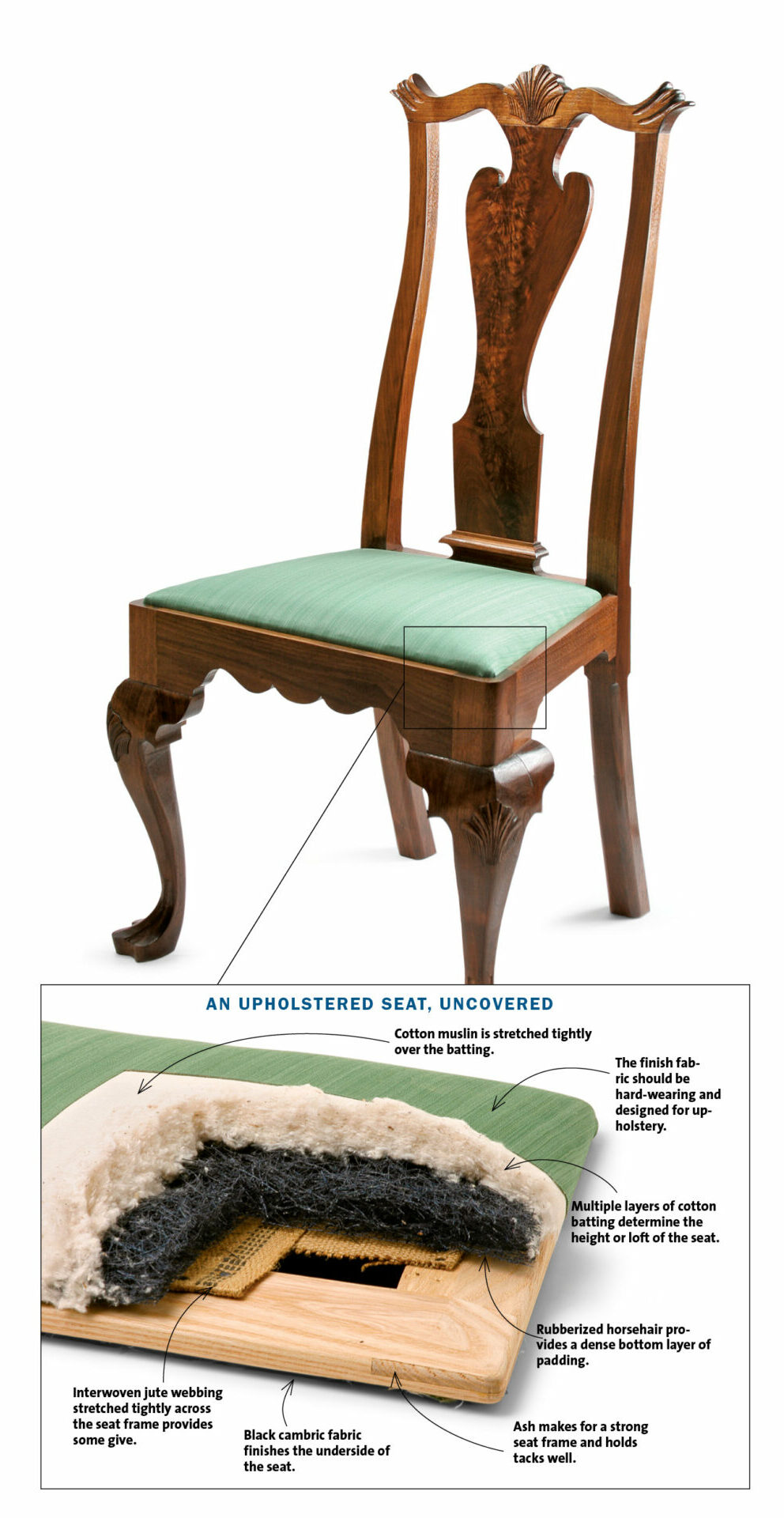This image combines a photograph and a diagram to thoroughly detail the construction of an upholstered seat. At the top, the photograph showcases a classic wooden dining chair with a dark, finely finished frame. The chair, noted for its vintage appeal, features ornate front legs and simpler back legs. A notable shell motif adorns the wooden backing, while the seat itself is upholstered in seafoam green satin. A small square highlights the front right corner of the cushion, connected by an arrow to the detailed diagram below. 

The diagram, titled "An Upholstered Seat Uncovered," dissects the seat's construction layers. It starts with an ash wood frame, renowned for its strength and ability to hold tacks well. Rubberized horsehair forms a dense bottom layer of padding, followed by multiple layers of cotton batting, which establish the seat's height and loft. Cotton muslin is stretched tightly over the batting, and the finished fabric, designed for durability, completes the surface. The underside of the seat is finished with black cambric fabric, while interwoven jute webbing, stretched tightly across the seat frame, provides additional support and flexibility. Each component is meticulously labeled and connected with arrows for clarity, offering an in-depth look at the craftsmanship involved in upholstering this elegant chair.